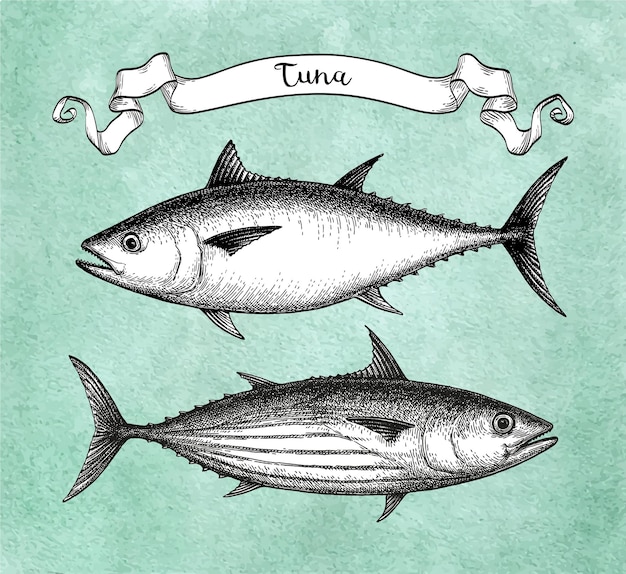The image is a flat, cartoon-style fish poster set against a light green, almost minty, watercolor-textured background. At the top of the poster is a classic, hand-drawn white banner with the word "TUNA" in prominent text. Below the banner are detailed, black and white illustrations of two different species of tuna. The top fish faces the left and has a stout belly, a sharp, long tail, and an open mouth. It is characterized by a very oval shape and spines along its top and bottom, with a crescent moon-shaped tail. The bottom fish faces the right, is darker with more shading, especially along the top half of its body, and has distinct horizontal stripes on its underbelly. Its fins and tail are similar to the fish above, long and sharp. Both illustrations are either hand-drawn or meticulously designed to appear as if they are, providing a clear and informative depiction of the tuna species. The overall layout is nicely framed and centered, ensuring a well-balanced presentation.